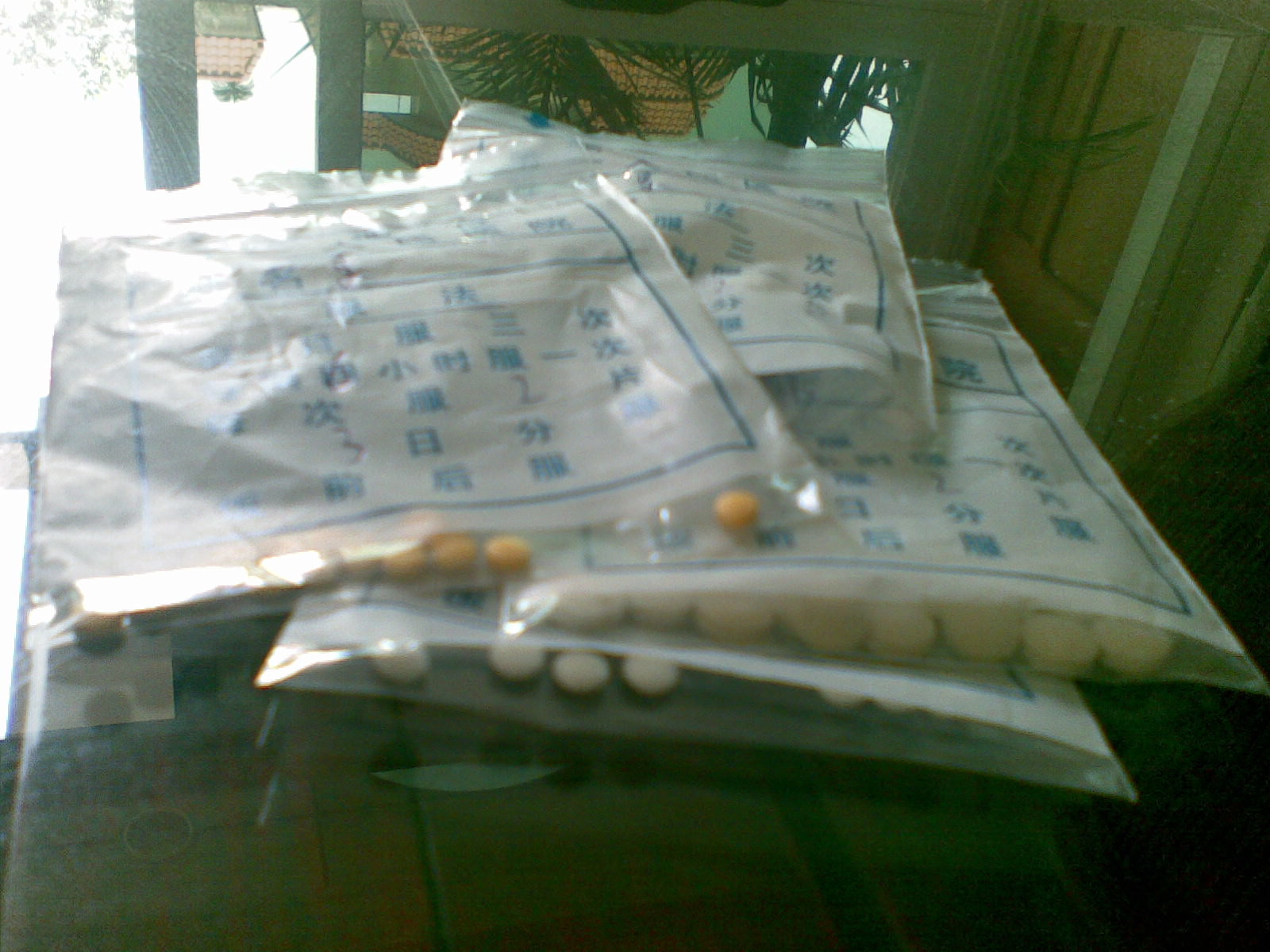This is a detailed photograph displaying four plastic ziplock bags stacked on top of each other on a glass surface tabletop. Each bag contains different types of pills; there are larger white tablets and smaller orange pills. The bags feature a piece of paper insert with blue rectangles printed with Asian characters, likely Chinese, suggesting the pills are of an Asian origin, possibly from Southeast Asia. The reflection on the glass surface reveals adobe-roofed houses, various palm trees, leaves, and an overcast sky, hinting at an outdoor environment visible from the room where the photograph was taken. The setting might be a pharmacy or a similar establishment. The image is very close-up, highlighting the details on the packaging and the pills themselves.